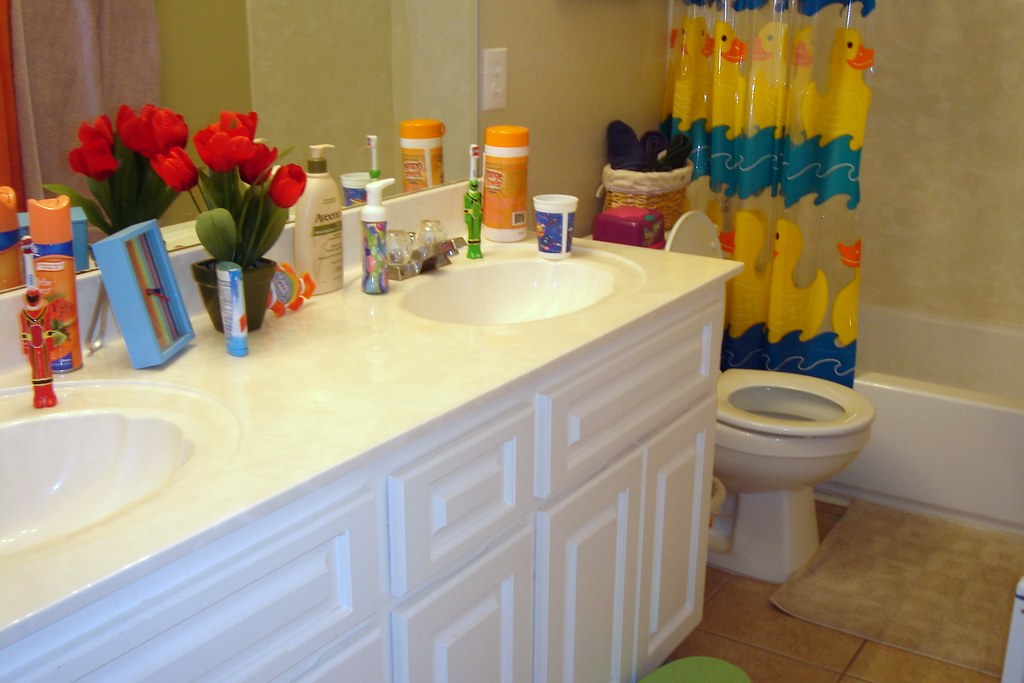In this image of a cozy indoor bathroom, the setting is highlighted by a pristine white cabinet with a white double sink vanity, both topped with an expansive mirror that reflects the room's features. The shower curtain catches the eye with its playful design of yellow ducklings swimming amidst blue water, the cheerful imagery set against clear vinyl material. The bathroom walls and floor are adorned in a rich brown hue, creating a warm and inviting atmosphere.

Central to the countertop between the sinks is a vibrant bouquet of red tulips, adding a splash of color and freshness to the room. The countertop also holds several practical items: a toothbrush, a blue rinse cup, a container of cleaning wipes, an air deodorizer spray, a tube of toothpaste, a dispenser of hand soap, and a bottle of hand lotion.

In front of the white toilet, which features a matching white seat, lies a soft brown rug that complements the tile floor. The thoughtful arrangement of elements in this bathroom creates a harmonious and welcoming space.